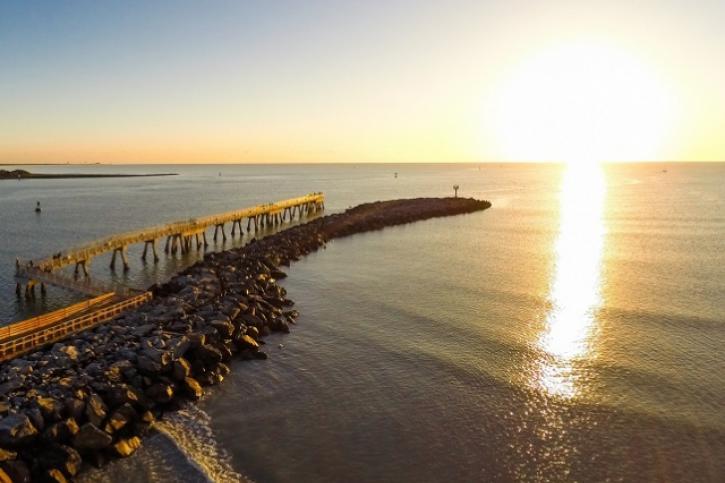As the sun sets on the horizon, casting a warm yellow reflection across the dark blue waters of the ocean, a serene and calming scene unfolds. The sky is clear, with hints of red near the horizon, and the ocean occupies about three-quarters of the image. To the left, a narrow, brown wooden wharf runs alongside an outcropping of black, jagged rocks that extend into the water, resembling a small peninsula. Waves gently crash against the rocks, adding a dynamic element to the otherwise tranquil scene. In the distance, a buoy floats, adding a minimalistic touch to the expansive seascape. The horizon is calm, with no people or boats in sight, emphasizing the peacefulness of the setting.